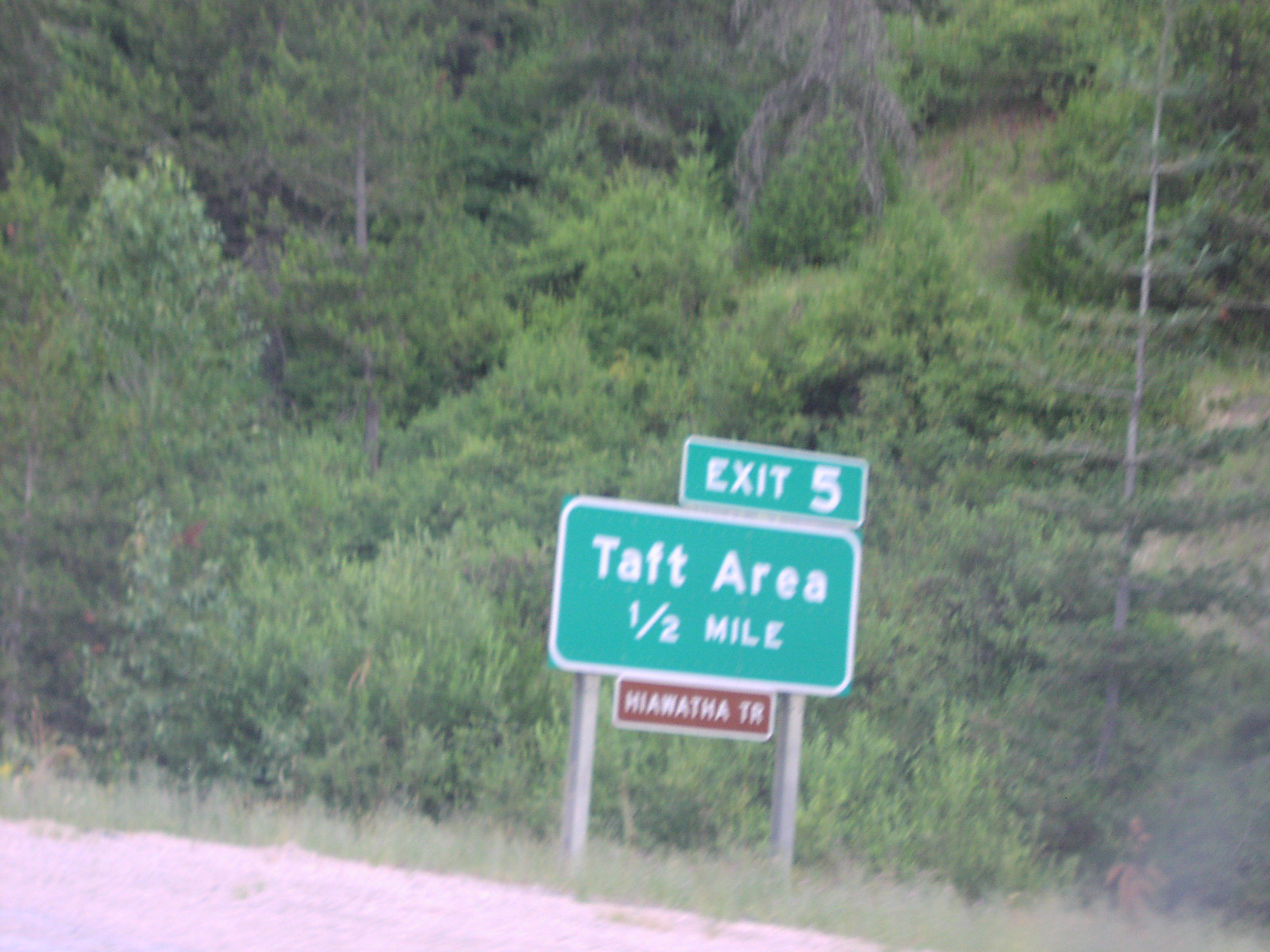The image captures a roadside scene set on an elevated stretch above a densely wooded area. The lush greenery of numerous trees dominates the background, creating a sense of depth and immersion in nature. At the center of the image, a turquoise road sign with a white border stands out strikingly against the verdant backdrop. The sign is divided into sections: the top part reads "Exit 5" in smaller, clear lettering. Below it, a larger segment displays "Taft Area, 1/2 mile," indicating the proximity of this destination. Further down, a section marked "Hiawatha Terrace" or potentially "Hiawatha TR," suggests specific directions or a local name. In the foreground, the ground is rocky and rugged, contrasting with the greenery that fills most of the frame, adding a textural variety to the scene.